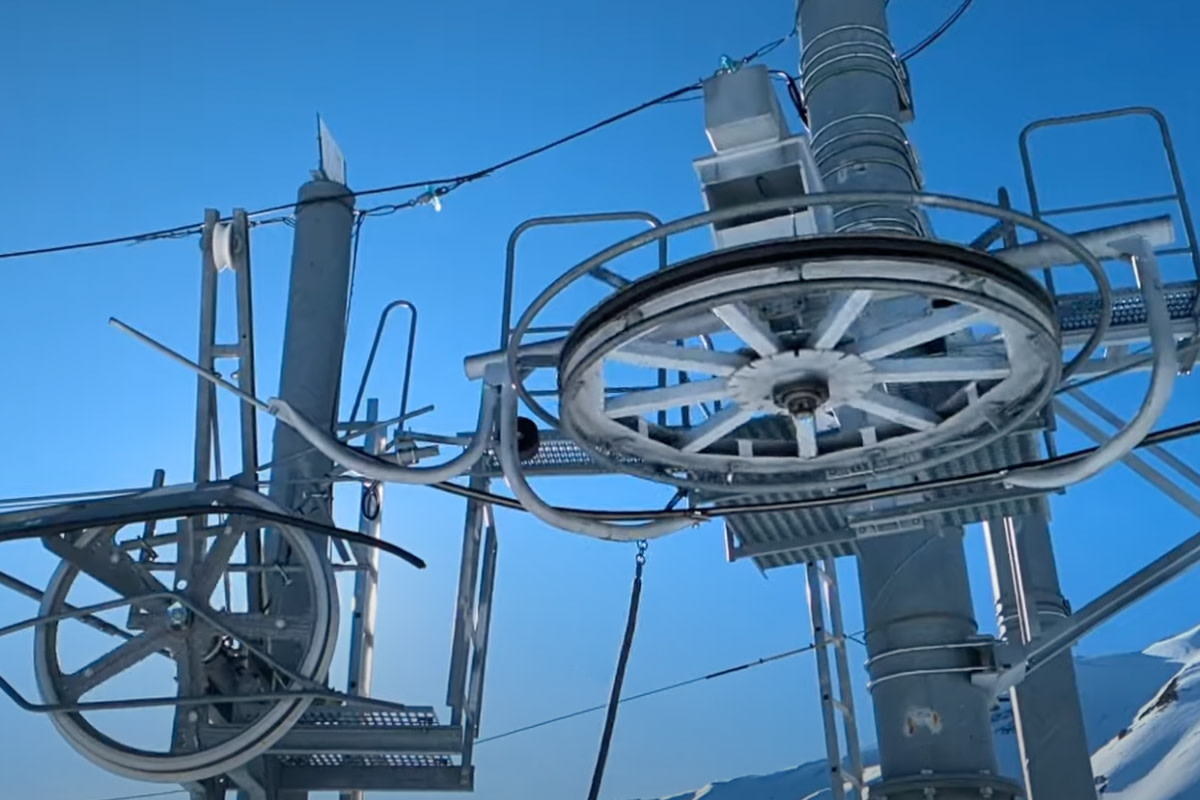The photograph captures the intricate contraption of a ski lift, showcasing its essential components against a wintery mountain backdrop. Prominently featured are two large round wheels: one positioned sideways and the other lying flat, both securely affixed to substantial metal poles. These wheels are enmeshed with various wires and framing, presumably functioning to rotate a cable that enables the lift's operation, allowing skiers to traverse the slope. The complex structure includes metal brackets, more wires, and additional metal grates with railings designed for maintenance purposes. The image is taken during the daytime, as evidenced by the light blue sky overhead and the sunlight glinting off the metallic surfaces. Snowy mountains can be seen in the background, specifically in the bottom right corner, emphasizing the cold, alpine setting of the scene. The overall color palette includes hues of sky blue, white, gray, and black.